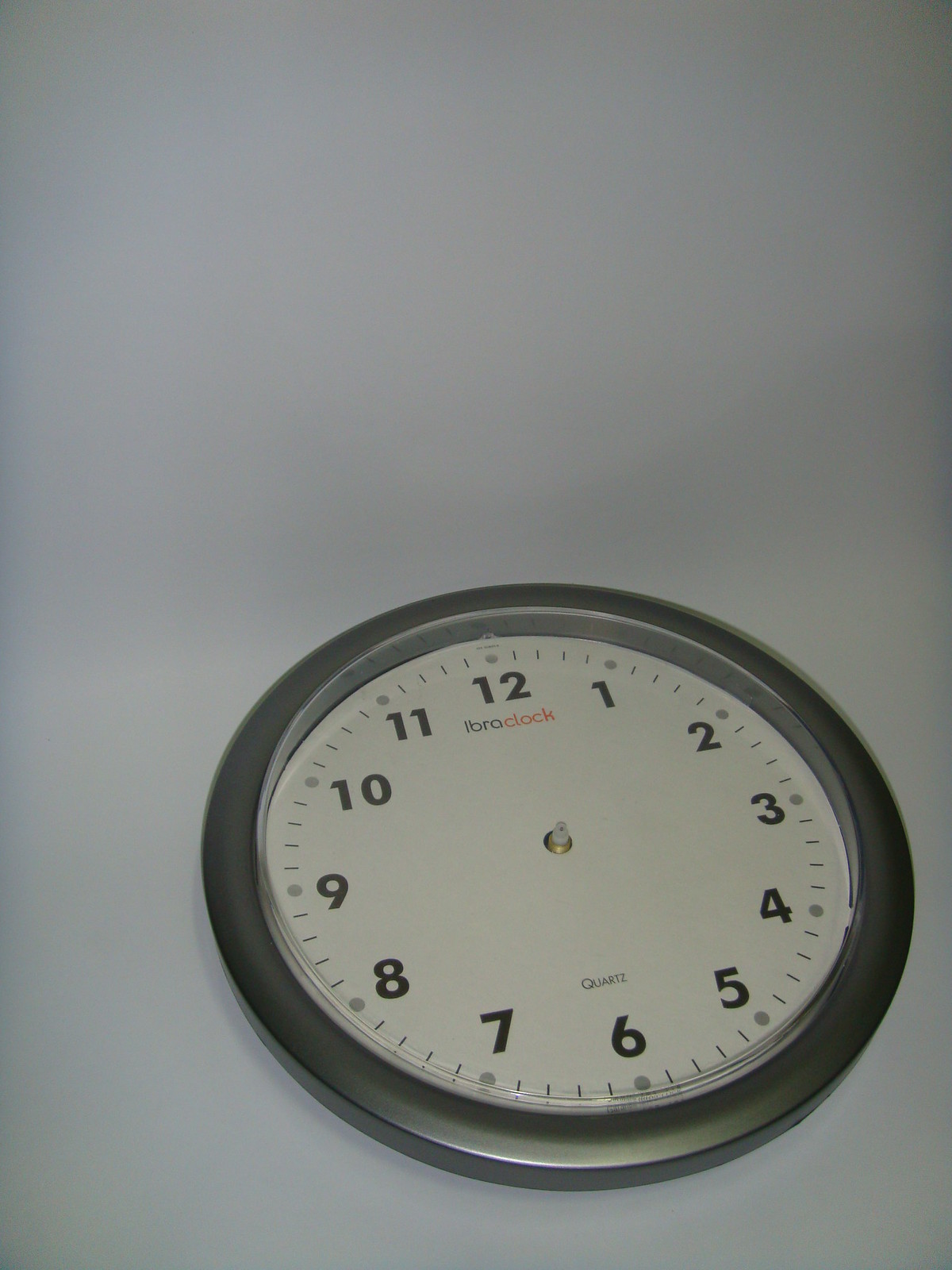The image depicts a clock taken from an angled perspective, slightly from below, likely causing some shadowing effects that give it an unclear background position. The clock is situated near the bottom right of the frame, where it appears to rest on a grayish surface with blackish tint near the top. The silver-rimmed clock, slightly tilted, shows the 12 positioned slightly to the left and the 6 to the right. It features a white face with black numerals in their usual order around the edge. Notably, the clock lacks hands. The brand name underneath the 12 reads "I-B-R-A clock" in black, followed by the word "clock" in red. Just above the 6, the word "quartz" is displayed in black lettering.